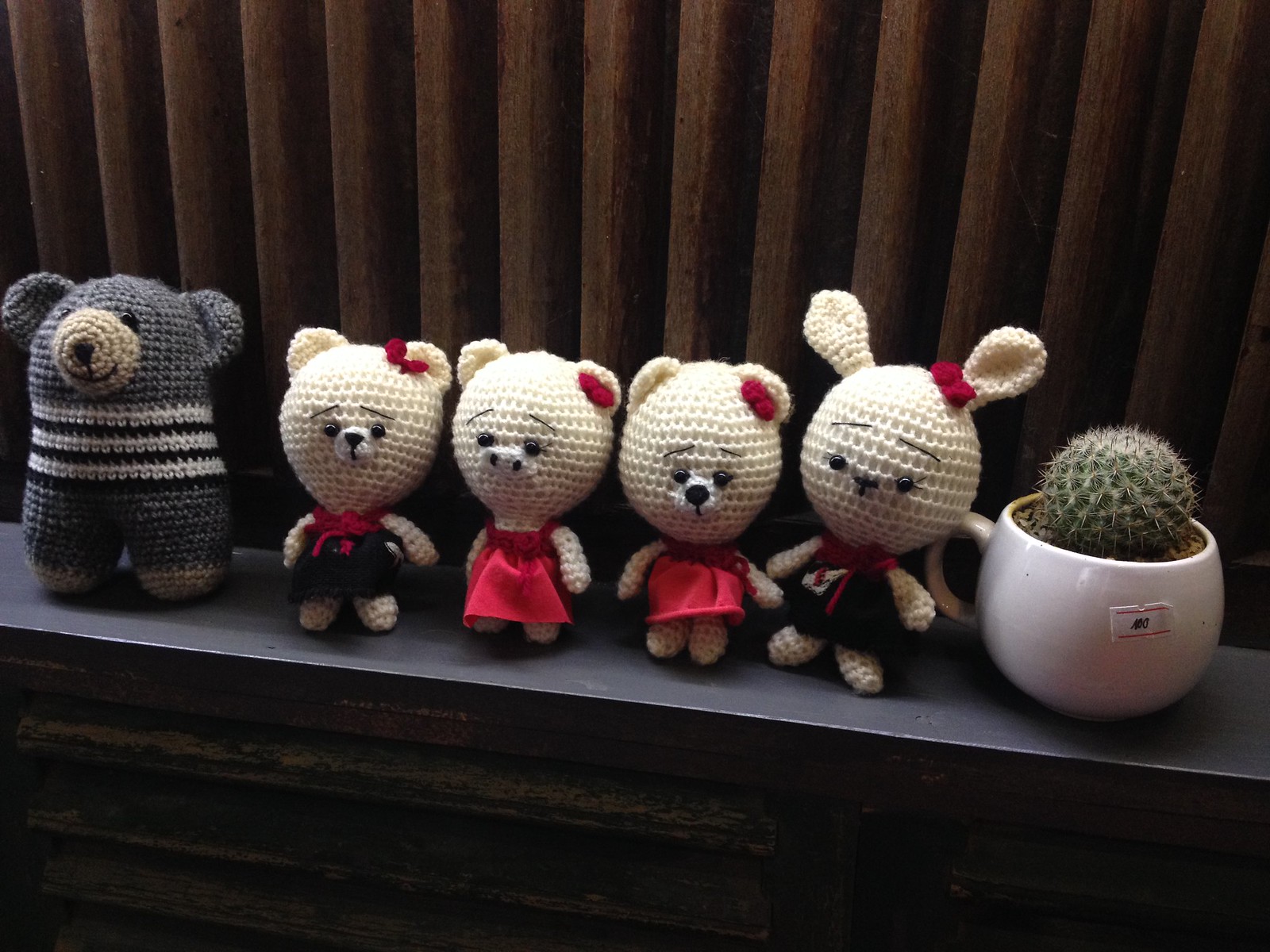On a gray windowsill with brown blinds in the background sit five charming crocheted animals and a cactus in a white mug. From right to left: a gray bear wearing a black and white striped scarf, sporting tiny ears, black eyes, a tan nose, and tan paws. Next, a white bear with a red bow near her left ear, wearing a sailor-like dress with a red top and black bottom. Following is a white pig with one red ear, raised eyebrows, and a snout, dressed in a red cloth dress. The third figure, another white bear, also features raised eyebrows and a red ear, donning the same red dress. Beside her, a taller white rabbit with asymmetric ears, a red bow, and a sailor dress consisting of a red top and blue bottom with a possible white pocket. Finally, a small spherical cactus resides in a dirt-filled white mug at the far left, adding a touch of greenery to the whimsical display.